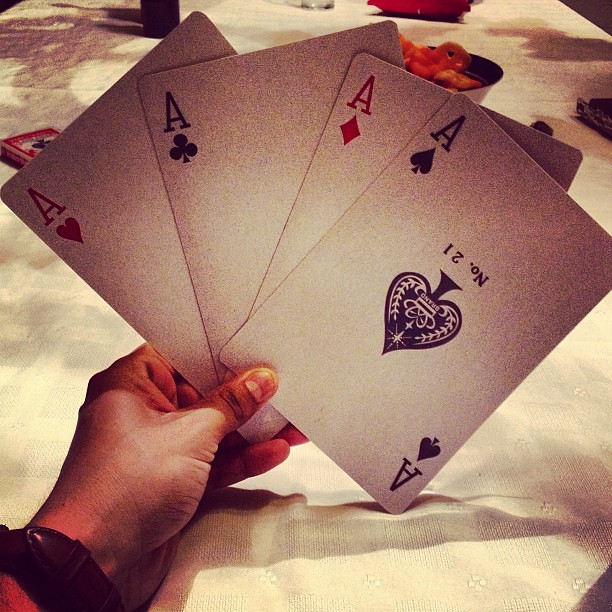In this evocative and slightly somber image, powerful contrasts of light and shadow frame a dramatic scene. Emerging from the bottom left corner, a hand adorned with a black leather wristband grips four oversized playing cards. These cards, arranged fan-like with the thumb in front, proudly display the aces of all four suits: from left to right, the ace of hearts, ace of clubs, ace of diamonds, and ace of spades. The detail in the hand's position adds a sense of tension and focus.

Set against a light tan tablecloth, the composition exudes a mysterious, almost cinematic atmosphere. In the background, toward the upper left, a predominantly red card box with black and white detailing lies partially in shadow, hinting at the origin of the cards. Further back, to the right, a bowl filled with cheesy puffs adds a casual, yet contrasting, element to the scene.

Shadow play enhances the overall mood, with distinct shadows cast by the hand and cards extending towards the right. This interplay of light and shadow infuses the photograph with depth and richness, drawing the viewer's eye across both foreground and background details.